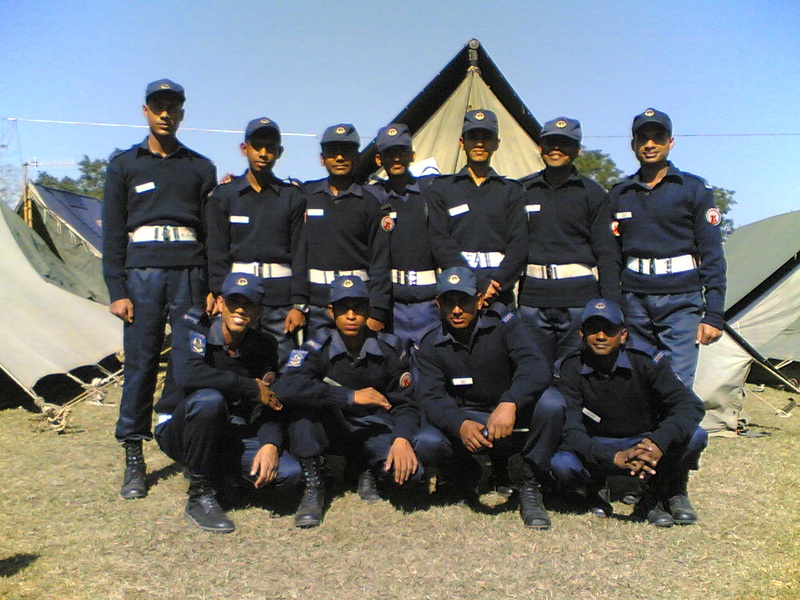In this detailed image, we see eleven dark-skinned men organized into two rows amidst a grassy field. The front row consists of five men kneeling, while the back row has six men standing. Each man is dressed uniformly in a navy blue long-sleeved shirt, with a collared shirt underneath, navy blue pants, black boots, and a navy blue hat adorned with a small, unreadable emblem. They also wear white belts and have patches on their shoulders, which are indistinguishable. Behind them are several tents in shades of blue, green, and beige, indicating a probable outdoor setting. The sky above is clear, contributing to a sunny atmosphere, and the men appear to be part of a military or police unit, suggested by their coordinated uniforms and name tags. The dry grass beneath them hints at a season outside of summer, likely late fall or winter.